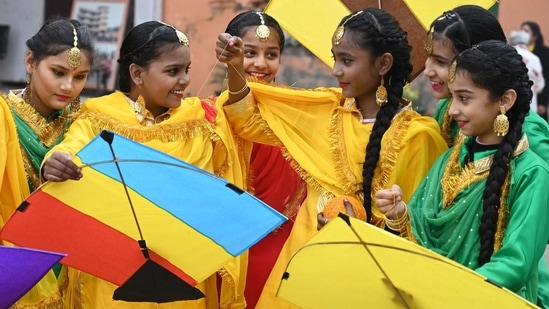This vibrant photo captures six young Indian schoolgirls, adorned in colorful traditional attire, standing outdoors in front of a wall, preparing to fly kites. Three girls on the left and middle are donned in striking yellow dresses, with the girl in the center donning a radiant red dress, standing just behind two of the girls in yellow. To the far right, two girls are wearing green dresses. Each girl is embellished with gold earrings and ceremonial headpieces that drape elegantly down from the middle of their hair to a medallion on their foreheads, emphasizing their cultural heritage. Their long hair is neatly braided, and their lips are accented with red lipstick. Notably, the second girl from the left proudly holds a kite with red, yellow, and blue stripes, while the girl on the far right clutches a solid yellow kite. Most of the girls are smiling joyfully, except for the one at the very left, who gazes downward with a serene expression. The girl's attire and accessories, including green accents and detailed emblems, reflect a harmonious blend of their traditional values and celebrations.